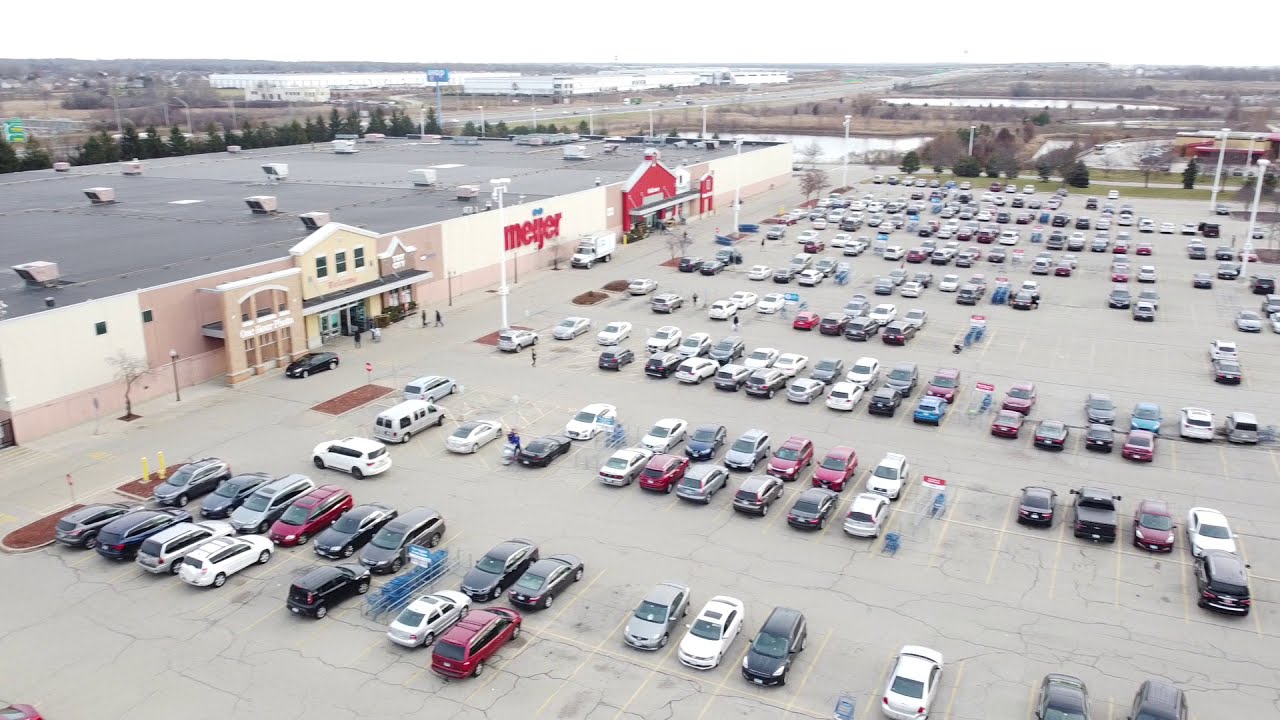The aerial photograph captures a bustling shopping center dominated by a massive, flat-roofed beige building labeled in bold red letters as "MEIJER," with distinctive blue circles positioned above the letters 'I' and 'J'. The expansive parking lot, which occupies the majority of the right side of the image, is filled with a diverse array of vehicles, including SUVs, four-door cars, and vans, indicating that more than half the spaces are occupied. Several metal racks for shopping carts are strategically distributed throughout the parking lot. In the scene, a prominent white box truck is parked in front of the Meijer store, which features a dark gray roof peppered with numerous white square vents and air conditioning units. To the left, additional store entrances are visible, leading toward the foreground of the image. In the background, the landscape includes a distant freeway and a large body of water, suggesting a Midwestern setting in the United States.